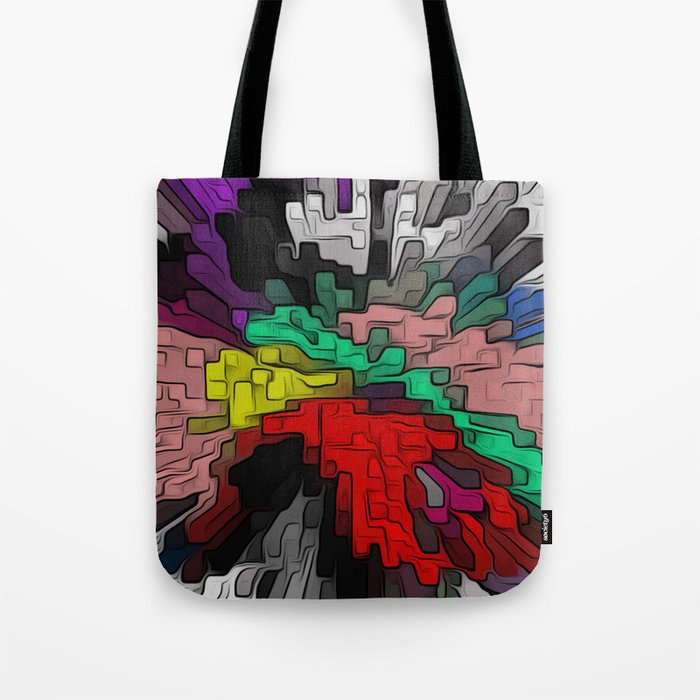This image is a close-up of a shopping bag set against a plain white wall. The bag features a black handle, but only the bottom part of the handle is visible as it attaches to the bag. The bag itself is strikingly multi-colored, displaying a vivid palette that includes purple, pink, green, yellow, red, blue, gray, white, and black. The design is highly impressionistic, appearing as though paint was dripped in square shapes that then spread out or melted, resulting in an array of irregular, overlapping squares. The overall effect gives the bag a dynamic, almost three-dimensional quality, reminiscent of an abstract painting.